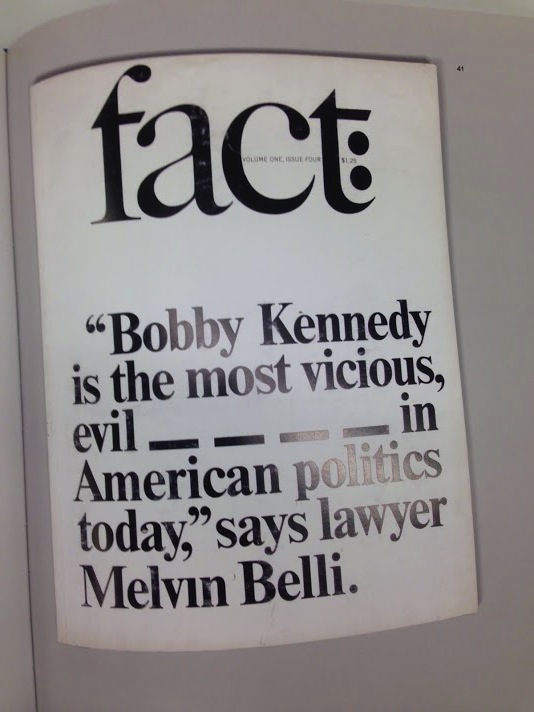The image features a vertically aligned rectangular display with a gray background, upon which a white piece of paper is positioned centrally. The paper appears slightly tilted to the left and has a curved look, as though it is lying on or attached to a curved surface. At the top of the white paper, in bold black print, the title reads "Fact: Volume 1, Issue 4, $1.25." Below this, the text, left-aligned, quotes lawyer Melvin Belli saying, "Bobby Kennedy is the most vicious, evil, ____ in American politics today," with four blank underscores suggesting a redacted or omitted word. The overall design of the image resembles a page from a publication or fact book, with the prominent quote aimed to grab the viewer's attention.